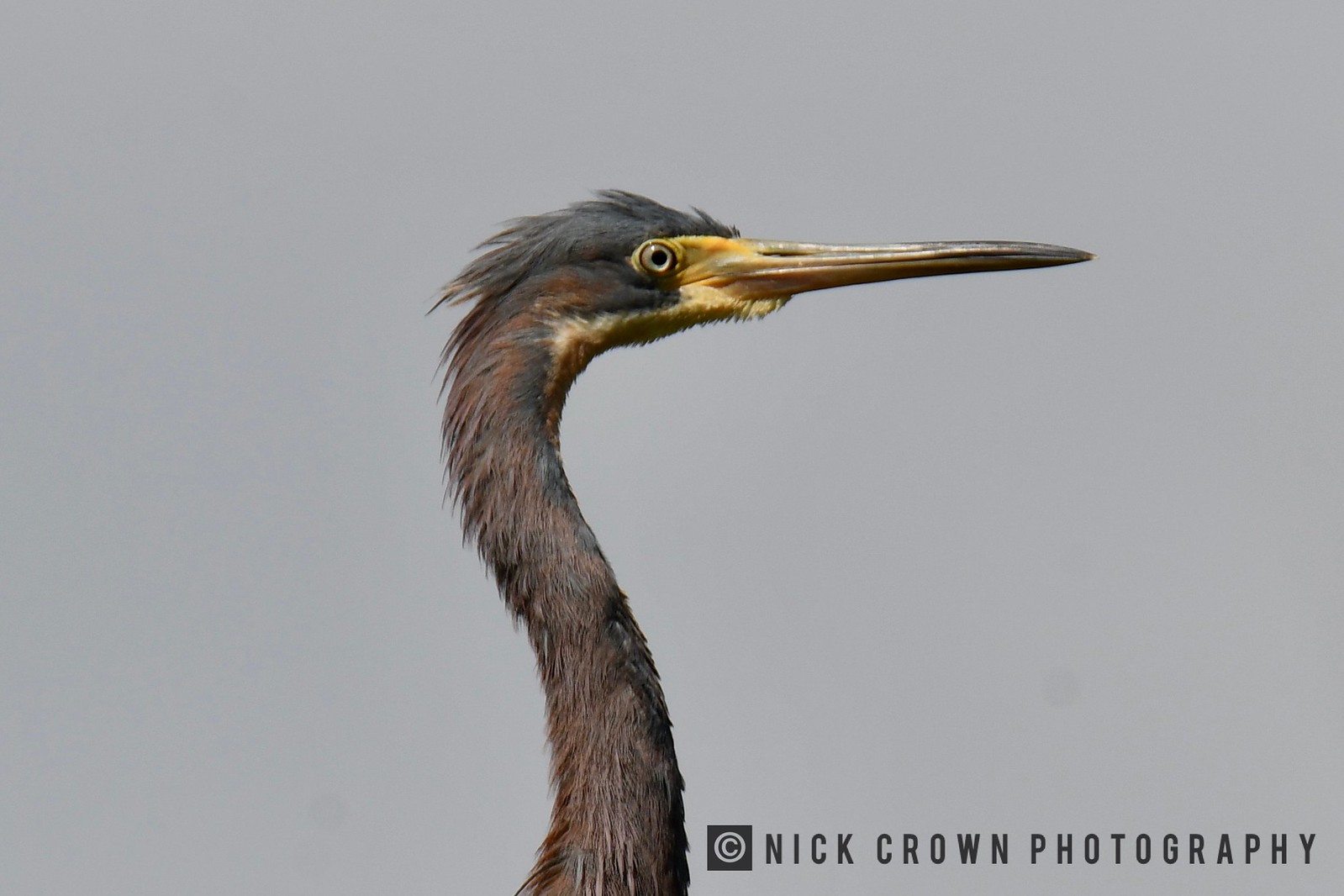The image features a single bird, centrally positioned, standing out prominently against a solid gray background. The bird, which is likely a large species akin to an ostrich or flamingo, showcases a strikingly long neck and a pointed, triangular beak. The beak is predominantly yellow with a darker, almost black tip, and a visible nostril. The bird's head has a small eye set in black feathers, while the neck is a contrasting mix of brown and tan hues, giving it a somewhat hairy appearance despite being feathers. No other objects are present in the image, enhancing the focus on the bird. The setting appears to be outdoors, captured professionally in daylight. In the bottom right corner, there is text that reads "Nick Crown Photography" accompanied by a copyright symbol.